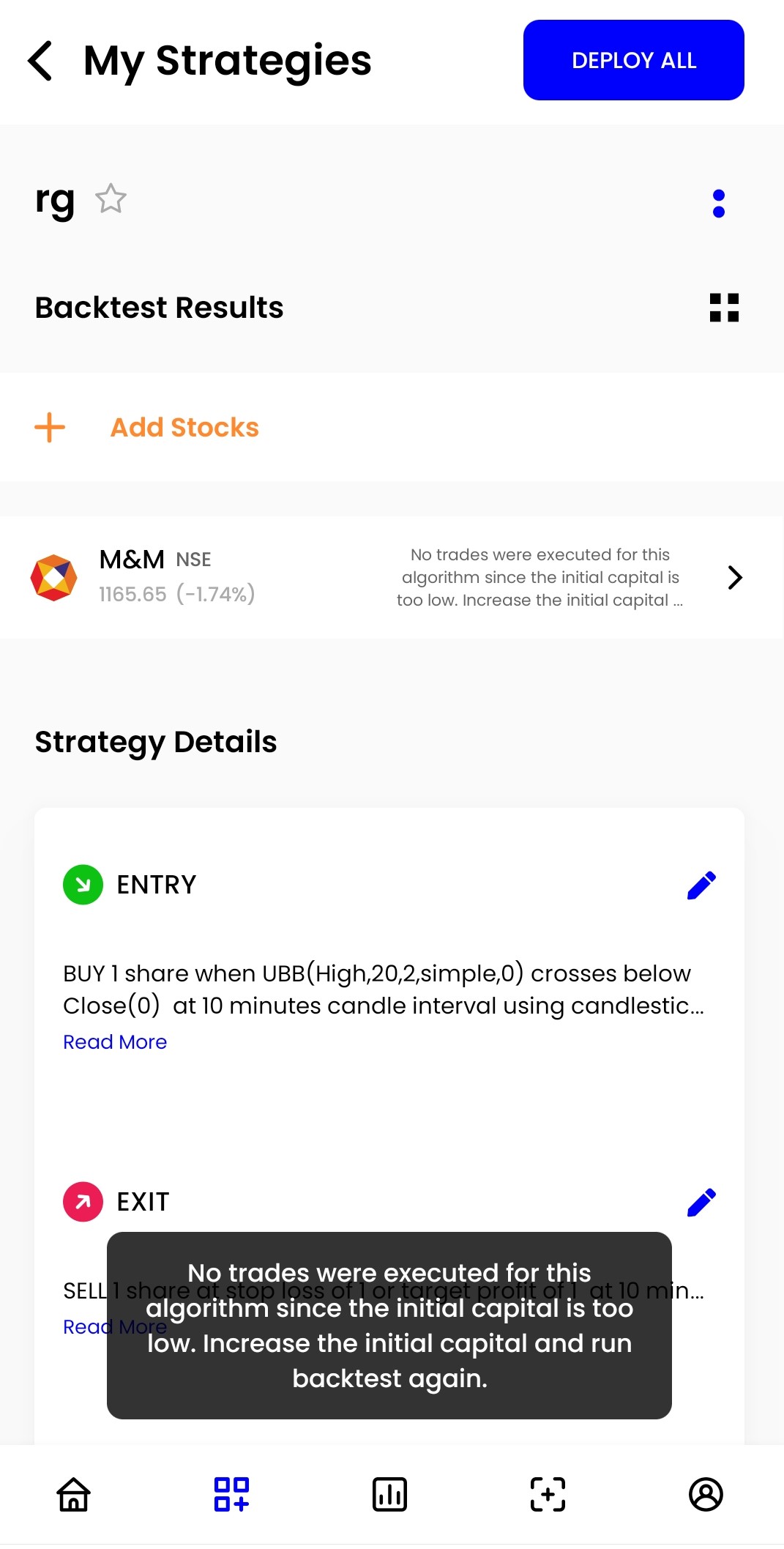This image is a screenshot from a smartphone displaying a webpage with a white background. The top part of the page is obscured, but visible elements include the header text "My Strategies" in black font, accompanied by a left-pointing arrow also on the left side. On the right side, there is a blue button with rounded corners labeled "DEPLOY ALL" in white, capital letters.

Further down on the left side, the text "Back Test Results" is visible, followed by an orange font link that says "Add Stocks," positioned next to an orange plus sign icon. Below this, the text "M&M" is displayed along with a light gray "NSE" label. To the left of "NSE" is an orange circular icon. 

The message "No Trades Were Executed For This Algorithm Since The Initial Capital Is Too Low. Increase The Initial Capital." appears in small gray font immediately beneath these elements. A gray rectangle with white font at the bottom reiterates the message: "Increase The Initial Capital and Run Back Test Again."

Within the main content area, the term "Entry" is listed, followed by a description "Buy One, Share One, UBB." Below this, "Exit" is mentioned, but the text is partially hidden by the aforementioned gray rectangle.

At the very bottom of the screen, there are navigation icons. On the right side is an icon indicating an account, and on the left side, there is an icon signifying a homepage.